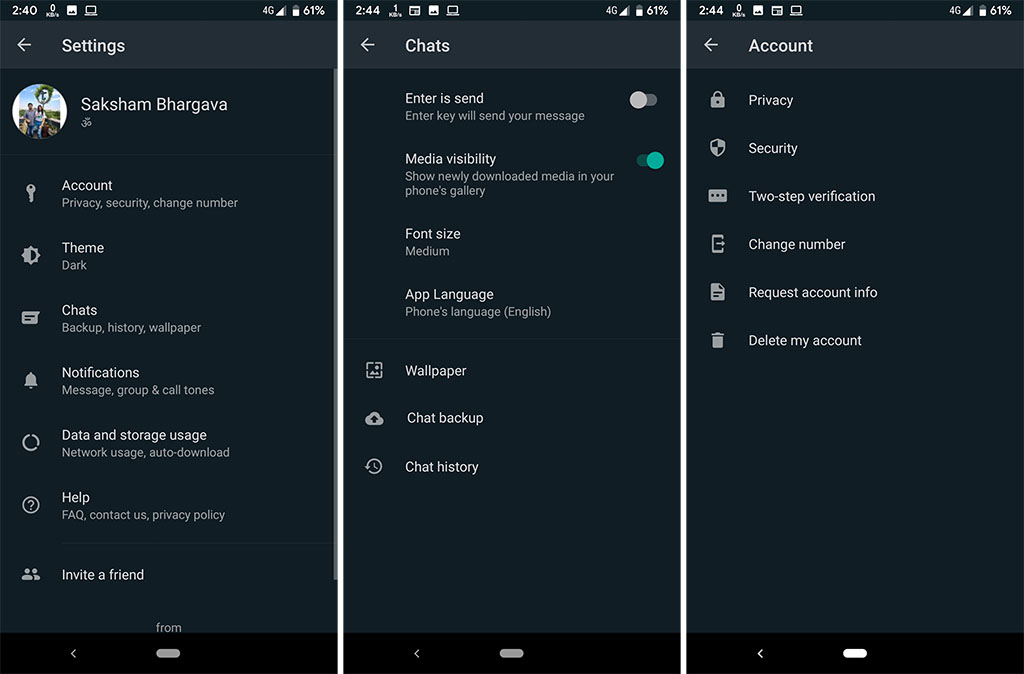This image comprises three distinct screenshots from a mobile device, ostensibly capturing sections of a chat application's settings, potentially WhatsApp, evident from the context. The trio of screenshots is time-stamped at 2:40 and 2:44 at the top of the screen.

**Left Panel: Account Settings Overview**

The leftmost screenshot showcases the user's account settings. At the top, it displays the user’s name, Saksham Bhargava, alongside a profile image. Directly beneath, a series of options are listed: 
- **Account:** 
    - Privacy
    - Security
    - Change Number
- **Chats:**
    - Theme (currently set to Dark)
    - Chats Backup
    - Wallpaper
    - History
- **Notifications:** 
    - Message, group, and call tones
- **Data and Storage Usage:**
    - Network Usage
    - Auto-download
- **Help:**
    - FAQs
    - Contact Us
    - Private Policy
- **Invite a Friend**

**Middle Panel: Chat Settings Specifics**

The central screenshot delves into the chat settings:
- **Enter is Send:** Switch toggled off
- **Media Visibility:** Switch toggled on
- **Font Size:** Set to Medium
- **App Language:** Same as the phone’s language
- Additional settings listed include: 
    - Wallpaper 
    - Chat Backup 
    - Chat History

**Right Panel: Additional Account Settings**

The rightmost screenshot reverts to more detailed account settings, presenting the following options:
- **Privacy**
- **Security**
- **Two-Step Verification**
- **Change Number**
- **Request Account Info**
- **Delete My Account**

This comprehensive analysis, indicating a messaging app’s settings page, suggests the screenshots could indeed be from WhatsApp, encapsulating key user settings.